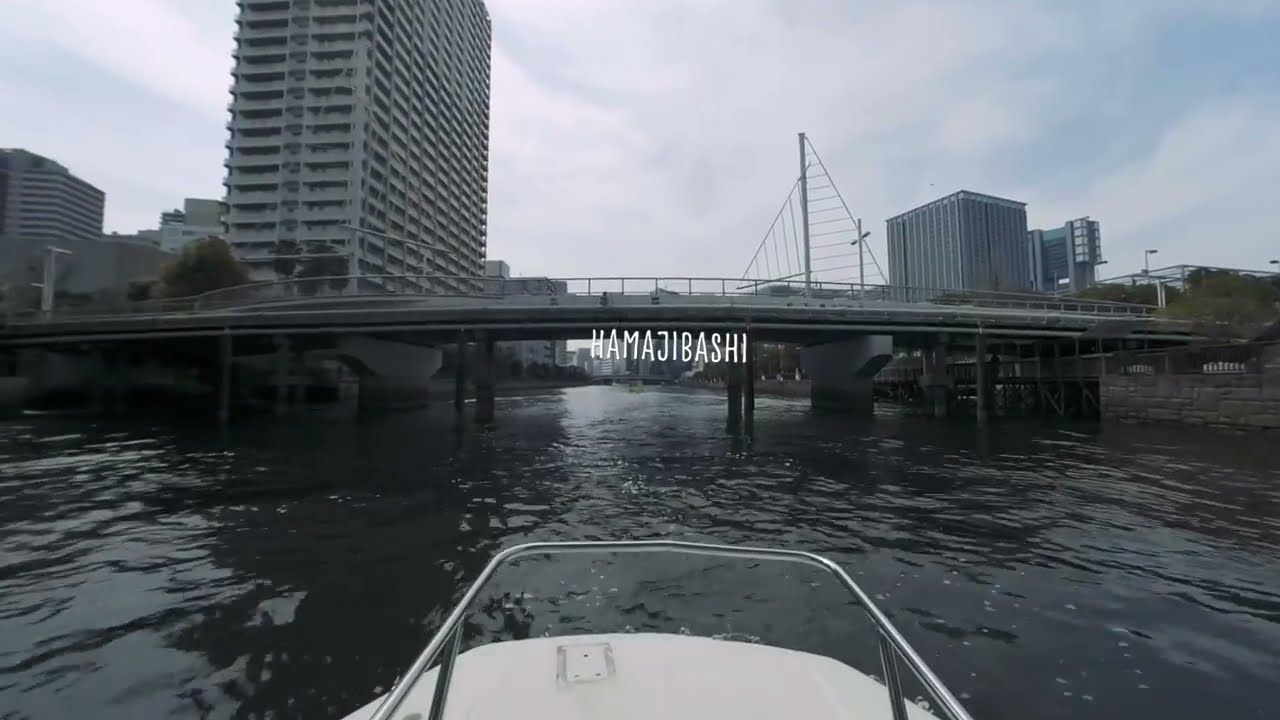This horizontally aligned rectangular image is taken from the perspective of someone on the front of a small boat, characterized by its silver railing and white front end, possibly with a window. The boat is navigating a body of water that looks like a grayish or dark green river, headed towards a small bridge about 50 feet ahead. The bridge is centrally positioned in the image, with the water flowing underneath it. Prominently displayed in white, all-caps text across the middle of the image is the word "HAMAJIBASHI."

Beyond the bridge, on the left side, stands a very tall high-rise building, soaring at least 20 stories, though it extends beyond the upper edge of the photo. To the right, there are several shorter buildings. Additionally, a unique structure resembling the wire frames of the sails and mast of a sailboat is visible on this side. These elements combine to depict part of a cityscape beyond the bridge, framed by gently rippling water in the foreground.